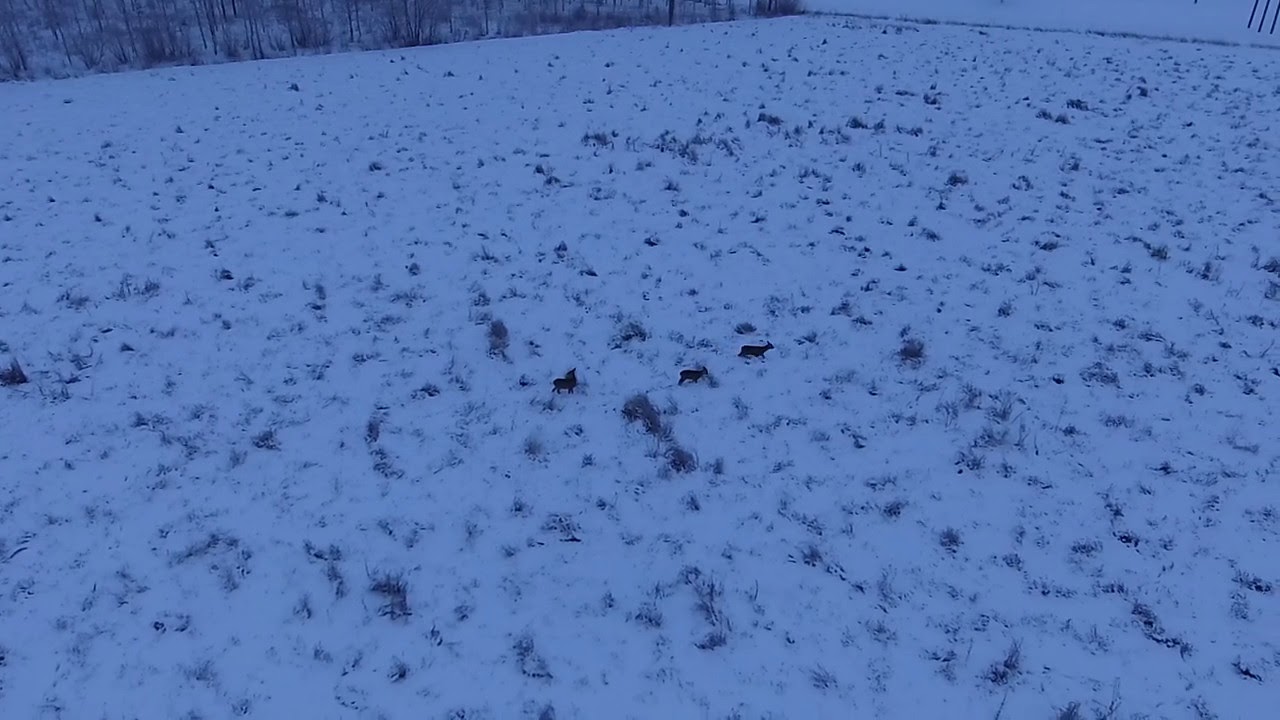The image depicts an aerial, bluish-toned view of a snow-covered field at dusk or night. The thin, slightly melted layer of snow reveals small patches and specks of grass and leaves beneath, creating a dotted appearance across the ground. Three black-colored animals traverse the field, their figures stark against the snowy backdrop. In the top left corner, thin trees are visible, while the rest of the field remains devoid of any significant structures, emphasizing the serene, open landscape.